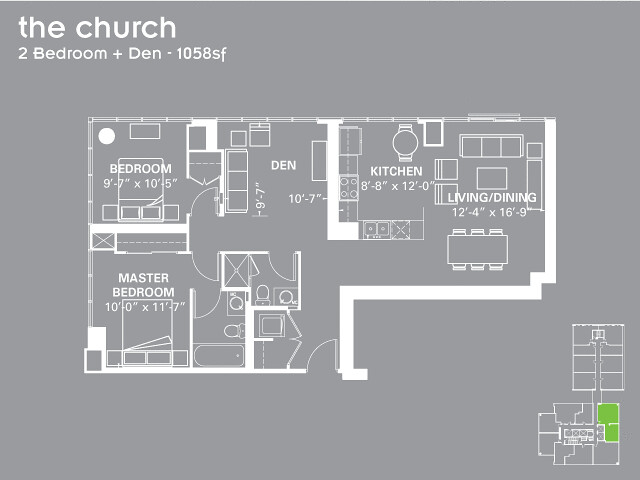This image showcases the detailed floor plans for a residential space described as "The Church," featuring a two-bedroom layout plus a den, totaling 1,058 square feet. The blueprint is meticulously rendered in white lines on a dark gray background, with the square footage prominently stated in the upper left-hand corner. Each room's measurements are clearly marked, including the two bedrooms, den, kitchen, living room, and master bedroom. The walls are depicted with both thick and thin white lines, emphasizing the structure's precision and computerized design. Door placements are indicated by curves that show the swing direction. In the lower right-hand corner, additional images are presented, possibly representing different levels or aspects of the house; one highlighted in green potentially suggests landscaping features. Despite the intricate detail, the only descriptor besides the layout itself is the title "The Church" at the top.